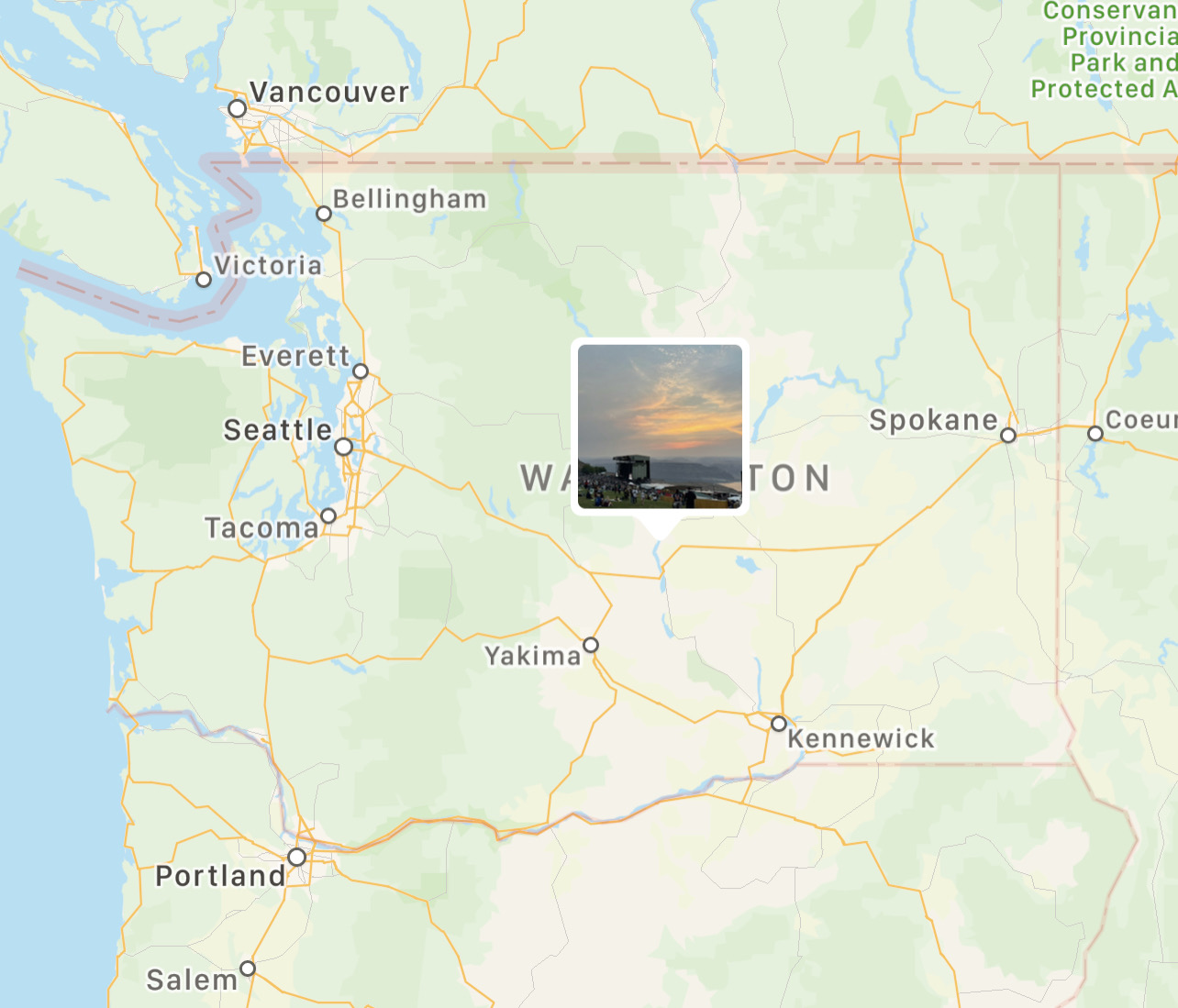The image is a close-up, full-color map of Washington State and its surrounding areas. It features varied coloration to denote different elevations and vegetation, with dark and light greens, yellows, and blues indicating bodies of water. Key elements include orange lines representing major highway routes and the placement of significant cities. Above the border with Canada, we find Vancouver, with Bellingham, Everett, Seattle, and Tacoma following southward. An island to the left highlights Victoria. In the central part of the state, below a small, framed photograph of a natural scene at sunset or sunrise, are Yakima and, further southeast, Kennewick. Spokane lies on the far right, near the top of the map. Beyond the Columbia River, near the bottom, the map marks Portland and Salem. There is also text in the upper right corner indicating "Conservan Provincia Park and Protected A," with the complete text partially off the image. The centerpiece photo, bordered in white, captures a scenic view over the ocean or mountainous landscape at either dawn or dusk, with a visible small building and some terrain.